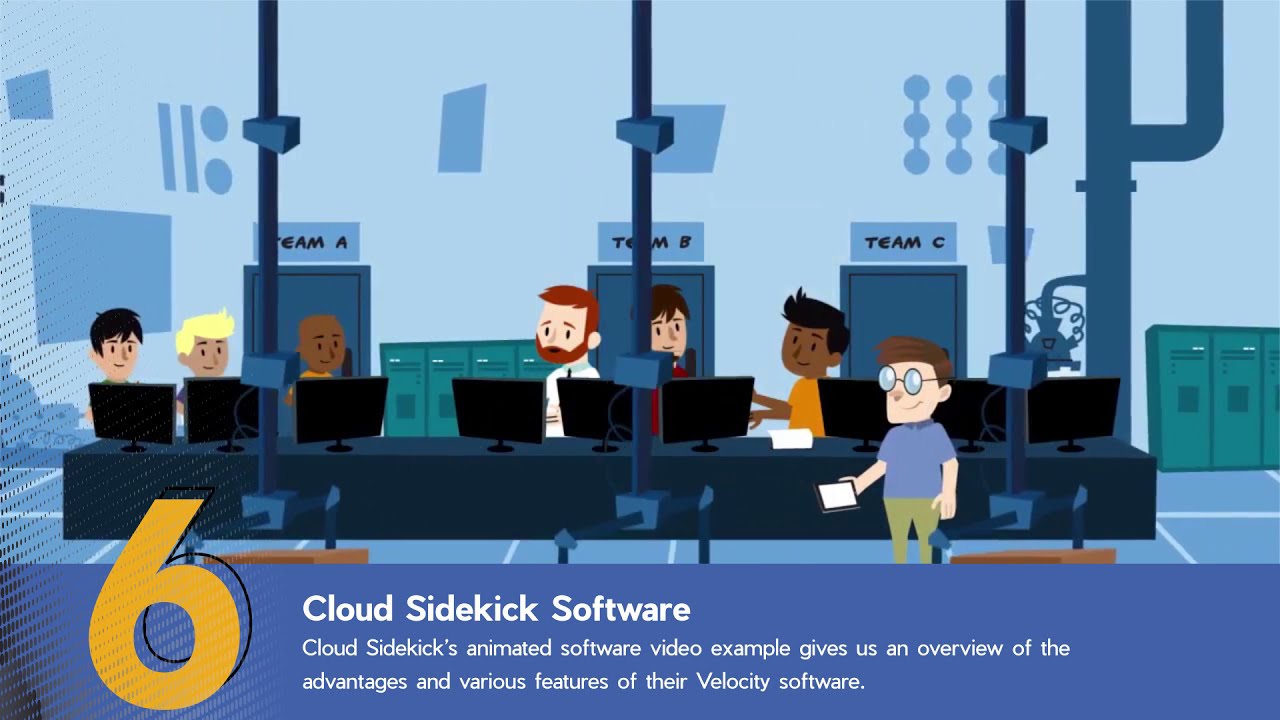In this animated digital art image, seven cartoon-like characters are depicted working in an office setting. They are gathered around a long blue table with black desktop monitors positioned in front of them. Six people are partially hidden behind the monitors, displaying diverse hair colors, such as brown, black, blonde, and red, as well as a range of complexions from lighter peach tones to darker browns. Visible clothing colors include orange, white, red, blue, and green pants. 

A smiling gentleman with glasses, wearing green pants, stands in front of the table holding a tablet. Behind the people, there are three doors labeled with banners: "Team A," "Team B," and "Team C." The background is predominantly blue, with green lockers situated between these doors and additional lockers on the far right along with what appears to be a pole or a pipe. 

Along the bottom of the image, a gold "6" is displayed, followed by a banner with white text on a blue background that reads, "Cloud Sidekick Software." The text, "Cloud Sidekick's animated software video example gives us an overview of the advantages and various features of their Velocity software," is also prominently featured, emphasizing the illustrative promotional nature of the image.